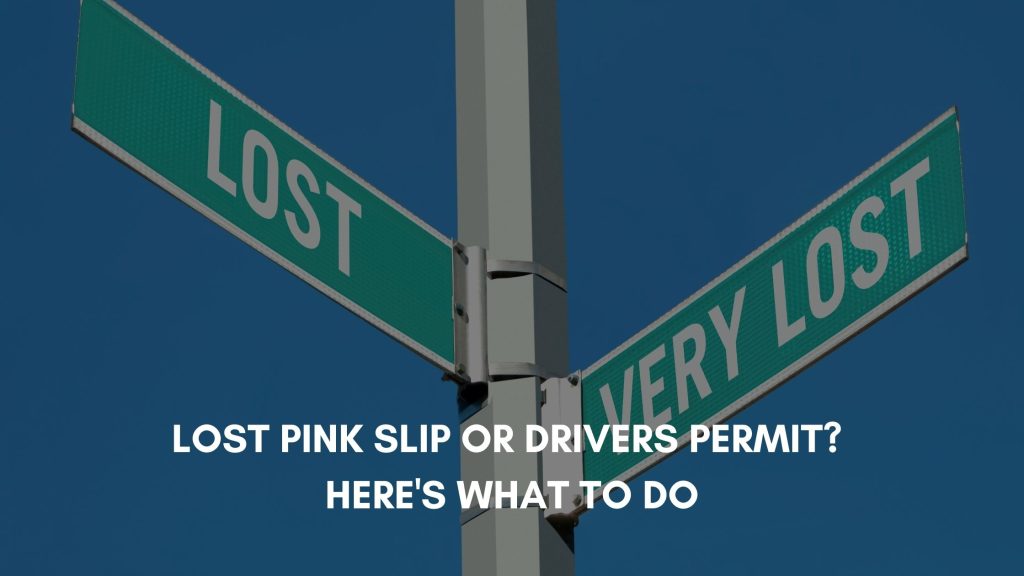In this computer-generated, stylized image set against an extremely blue background, a vertical metal signpost stands prominently, adorned with two green street signs. The sign on the left reads "Lost" while the one on the right says "Very Lost," both in white lettering. Below these street signs, a white-text overlay reads: "Lost Pink Slip or Driver's Permit? Here's What to Do." The overall color scheme features subdued blues, greens, and grays, making the white text pop against the darker tones. The setting evokes an amusing sense of direction (or lack thereof), serving as a visual metaphor for providing guidance on replacing important documents.